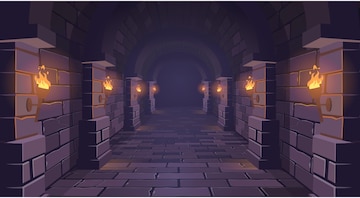This computer-generated image depicts a dark, dungeon-like hallway reminiscent of a passageway in a castle or catacombs, often found in fantasy settings like video games or illustrated books. The hallway is constructed from large, gray stone blocks that form both the floors and walls, giving it a very structured, almost cartoony appearance. Along the walls, there are four brick pillars on each side, each adorned with a brown sconce holding a lit torch. The sconces, eight in total, emit an orange-yellow flame, providing the sole illumination in the otherwise very dark environment which features hues of purple and black. The ceiling arches gracefully in a curved shape, contributing to the overall immersive and foreboding atmosphere. The hallway fades into darkness, adding to its mysterious allure. It’s a meticulously crafted digital illustration with no text or individuals present, further emphasizing its eerie and deserted nature.